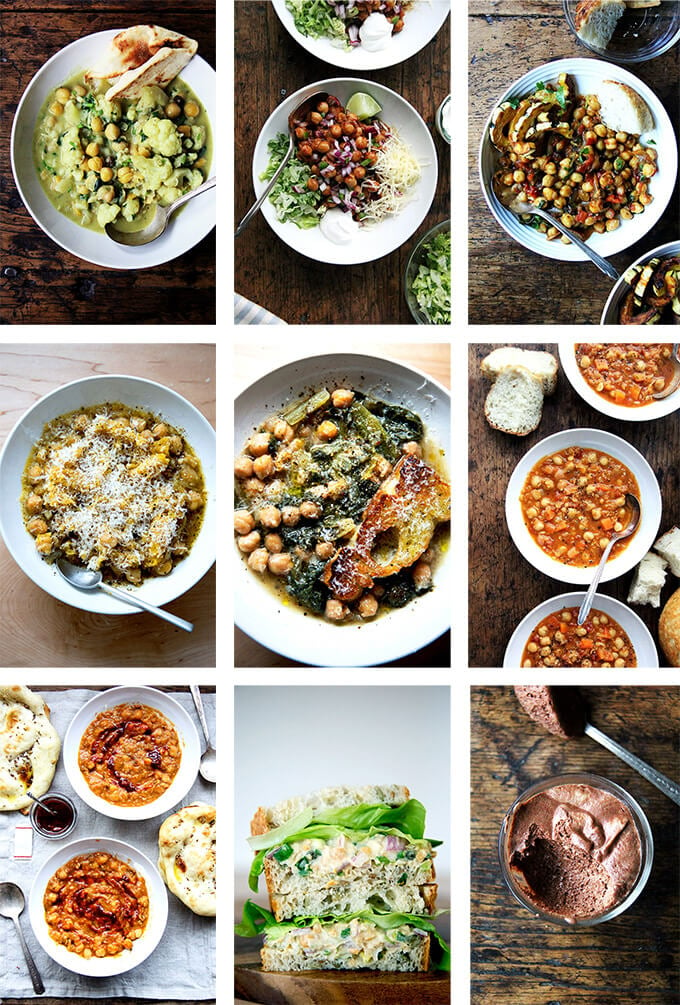This is a visually rich diagram consisting of various photographic images of food dishes, meticulously arranged in a magazine spread-like grid. Central to most of these dishes are chickpeas, also known as garbanzo beans, which are featured in diverse culinary forms, emphasizing their versatility. 

On the left-hand side, chickpeas appear in a green soup, accompanied by hummus and a light bread slice. Moving to the center, chickpeas are seasoned, possibly with a brown bread seasoning, and another central image showcases chickpeas topped with cheese. A further dish features chickpeas with vegetables and garnish, enhanced by a piece of golden-brown bread.

On the right side, there are three bowls of chickpea soup, identifiable by their yellow chickpeas amidst a red, possibly tomato or spice-based broth, each with a piece of cut bread positioned near it. The bottom section reveals a variety of dishes; a brown dessert in the lower right, and a layered bread dish filled with garnish in the center. Additionally, two bowls spiced with dark red chili sauce are placed in the lower left, with cooked bread and a spoon visible.

The images predominantly use white round dishes, set against a dark background, creating a vivid contrast that highlights the bright colors of the food. The rustic, possibly international cuisine, features chickpeas prominently, alongside green lettuce, sprouts, cheese, and varied breads, showcasing a multitude of chickpea-based culinary possibilities.